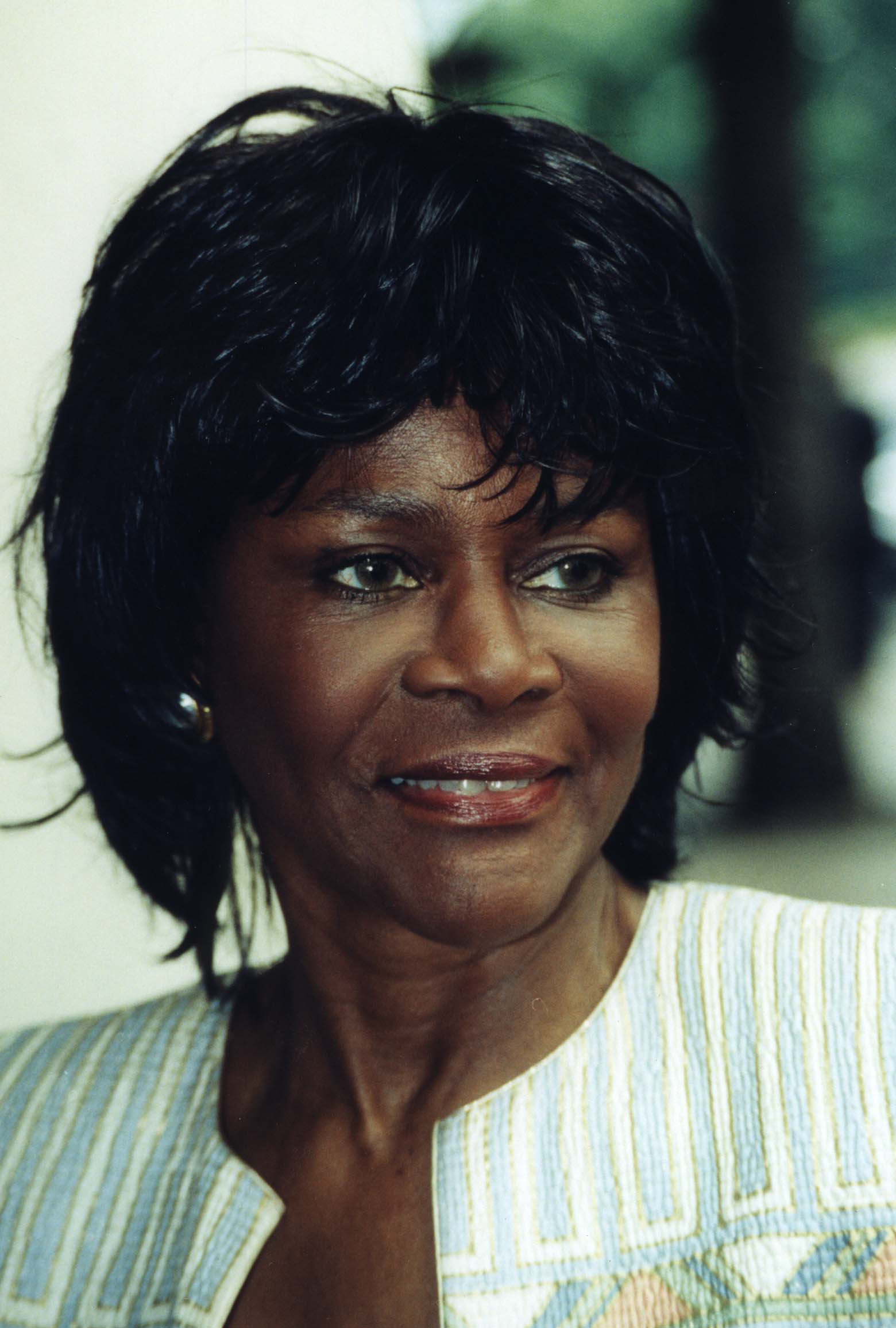The photograph captures a close-up of a smiling black woman, possibly in her late 50s to 60s, only visible from her upper shoulders to the top of her head. She is gazing towards the right side of the image. Her shoulder-length, slightly wavy, jet-black hair frames her face, with some strands falling near her eyes. She wears bold red lipstick and large gold circle earrings with silver caps, the right earring prominently visible. She is dressed in a blue and white striped top adorned with various geometrical designs in blue, green, and orange. The background is out of focus, featuring large black trees with green leaves, enhancing the emphasis on her vibrant appearance.